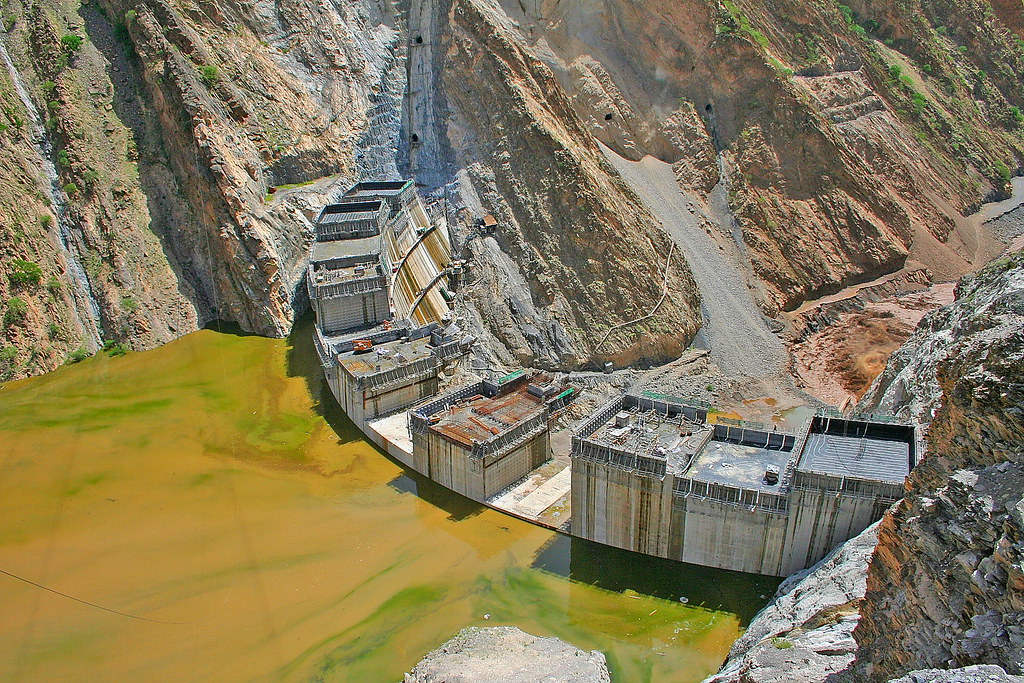This detailed aerial landscape photograph captures a small, old, and rickety mining community nestled along the side of a rocky hill, framed by a partially constructed dam. The scene is set in a rugged, steep terrain devoid of snow but filled with ominous rocks and scarce greenery. Behind the waning rows of ancient buildings, possibly warehouses with no visible windows or roads, lies a distinctive, murky, and heavily polluted lake marked by stagnant, mustard-colored and greenish-brown water with streaks of algae.

The backdrop showcases a series of towering, gray-black mountain rocks, threaded intermittently with trees and punctuated by tunnels burrowing into the rocky facade. Much of the valley appears extensively excavated, revealing the dam composed of large, uneven box-like concrete sections, some level with the murky waters and others jutting prominently above it. The bottom of this scene is characterized by a muddy gravel pit road, winding upwards towards these caves within the rock. The dam itself curves gently, its higher sections showing signs of ongoing construction, forming an arc with a dry spillway on its right side and polluted waters pooled to its left. The overall atmosphere is oppressive and sere, making it seem like a desolate and inhospitable place.